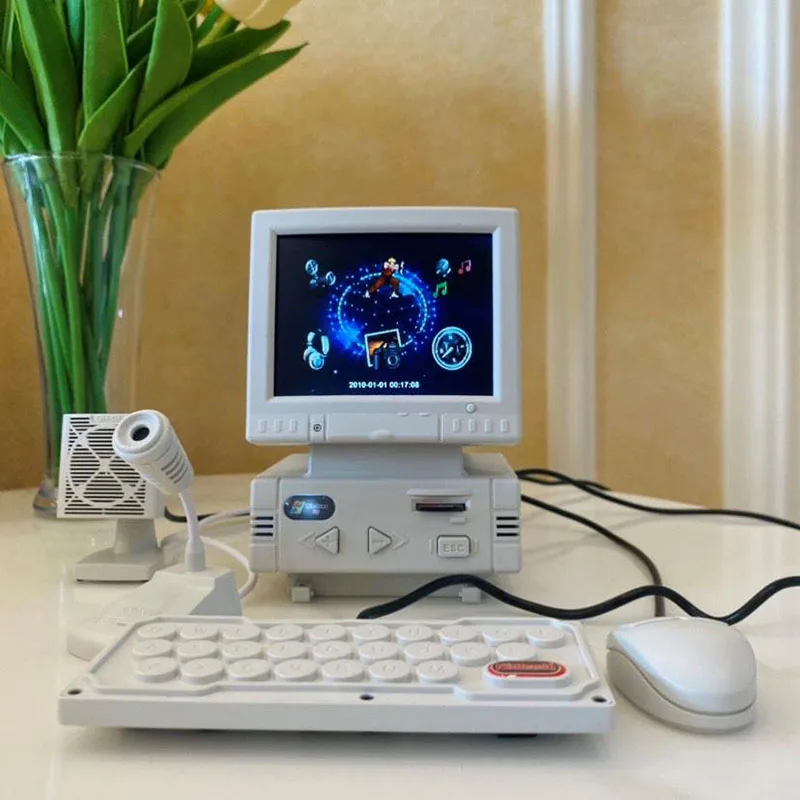The image depicts a miniature toy computer setup on a white table positioned against a beige wall with white molding. The table is adorned with a clear vase containing green plant stems and a partially visible white flower, possibly a tulip, on the left side. The main focus is a small, old-style computer setup featuring a plastic CRT monitor and desktop computer. In front of the monitor lies a small, white plastic keyboard and a corded white mouse, plugged into the keyboard itself. Positioned to the left of the computer are an old-style white microphone and a white fan or speaker. The computer screen displays a blue orb and other small, unclear images, while the computer front is designed with two arrow buttons and what appears to be a fake disk drive and an on-off switch.